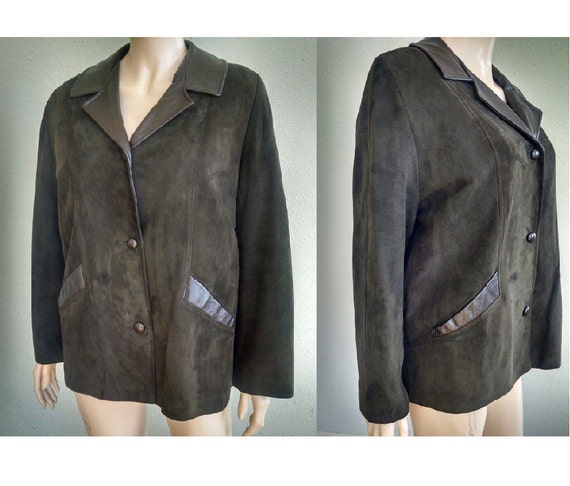The image consists of two photographs of a dark suede jacket on a cream-colored mannequin, set against a light green background. The mannequin's torso, arms, and legs are visible, but its head is out of frame. This jacket, which may appear either green, gray, or brown, has wide lapels and is buttoned down the front with three buttons. The jacket features leather accents, including a prominent, large leather collar, and reflective material above the pockets, which adds a lighter, shiny contrast to the garment’s overall dark hue. The left photograph captures the mannequin facing straight at the camera, while the right photograph shows the mannequin angled to better display the side view of the jacket. The jacket appears slightly worn, suggesting it might be second-hand, likely being showcased for an online sale.